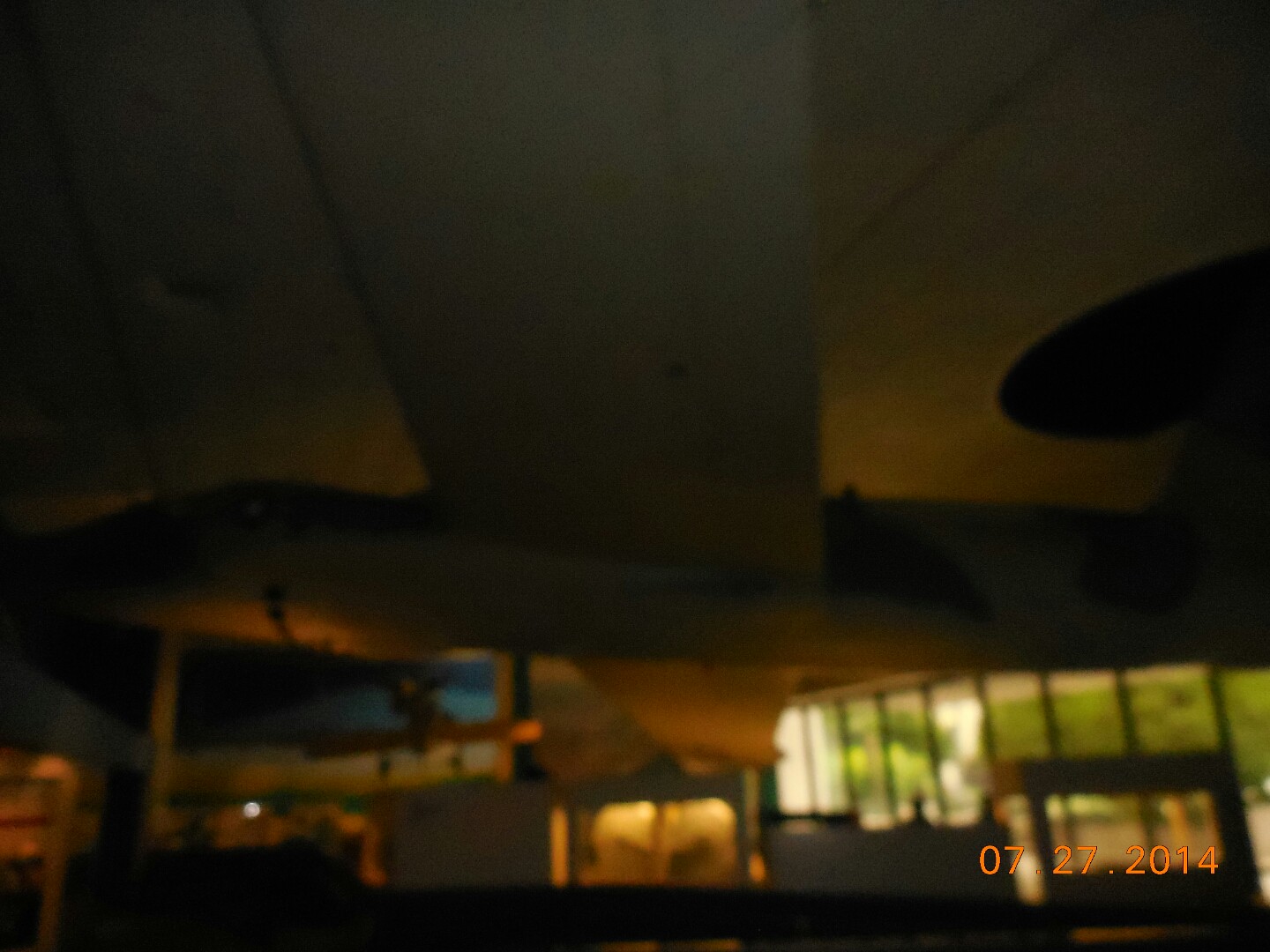This blurred image, dated 07/27/2014 in the bottom right corner, depicts a room characterized by floor-to-ceiling windows along the bottom left side, showcasing a glimpse of greenery outside. These windows are the primary light source in the room. The ceiling appears to be made of concrete and features an additional wide, protruding section that spans halfway across the space. A light fixture, embedded within this protruding section, casts a limited glow and creates subtle shadows on the ceiling. Various pieces of furniture are partially visible beneath, including a table with an illuminated area underneath it.